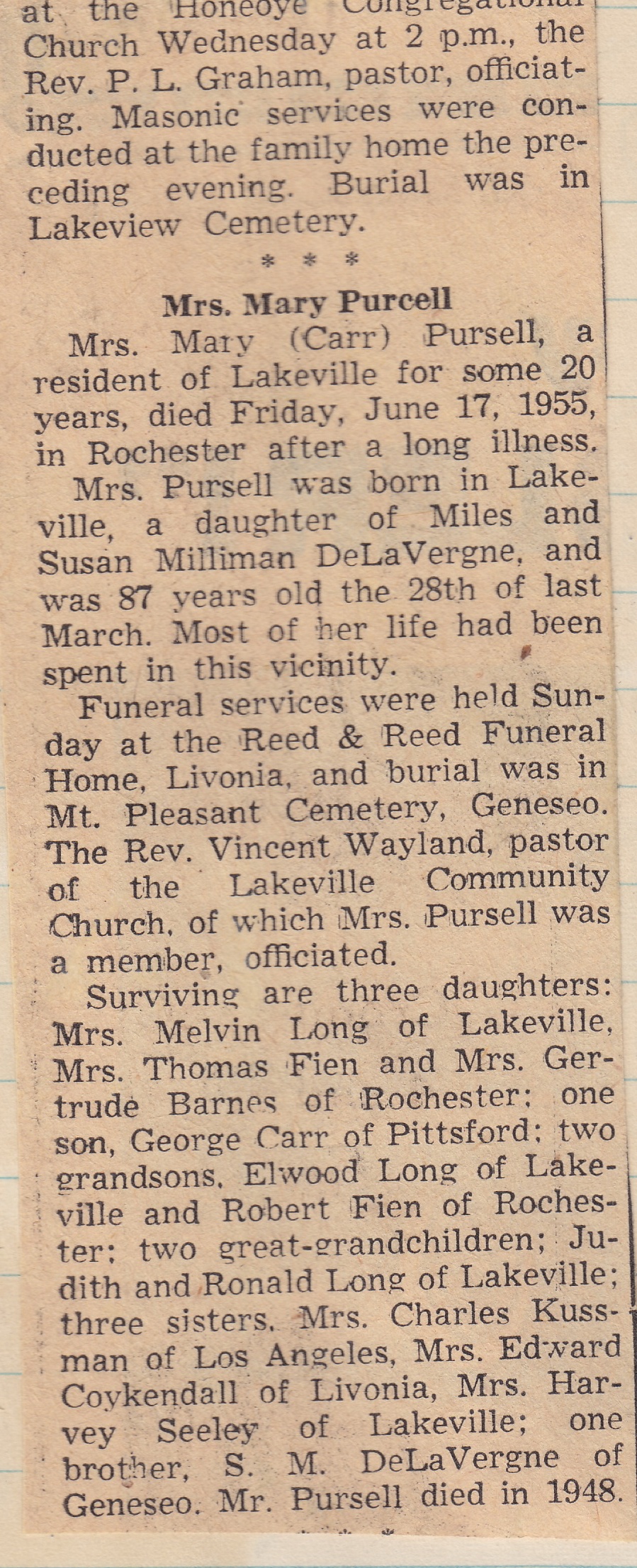The image is a photograph of a yellowed and faded newspaper obituary for Mrs. Mary Carr Purcell, a long-time resident of Lakeville who passed away on Friday, June 17, 1955, in Rochester after a prolonged illness. Born in Lakeville as the daughter of Miles and Susan Milliman de la Verne, Mrs. Purcell had reached the age of 87 on March 28 of that year. The obituary details her local ties and the significant portion of her life spent in the vicinity. Funeral services took place on Sunday at the Reed and Reed Funeral Home in Livonia, with burial at Mount Pleasant Cemetery in Geneseo. The services were officiated by Reverend Vincent Wayland, the pastor of the Lakeville Community Church, where Mrs. Purcell was a member. She is survived by three daughters: Mrs. Melvin Long of Lakeville, Mrs. Thomas Flynn, and Mrs. Gertrude Barnes of Rochester; one son, George Carr of Pittsburgh; two grandsons, Elwood Long of Lakeville and Robert Fien of Rochester; and two great-grandchildren, Judith and Ronald Long of Lakeville. Additionally, she leaves behind three sisters: Mrs. Charles Kussman of Los Angeles, Mrs. Edward Kuykendall of Livonia, and Mrs. Harvey Seeley of Lakeville, as well as one brother, S.M. de la Verne of Geneseo. Her husband, Mr. Purcell, preceded her in death in 1948.